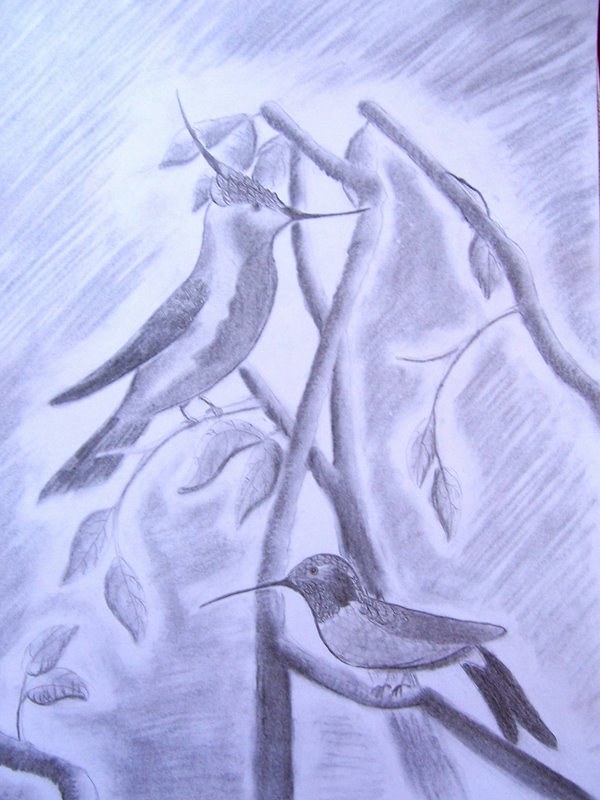The image is a detailed pencil or charcoal drawing on a white piece of paper, depicting an intricate scene of two birds perched on overlapping twigs. The twigs cross in an X pattern in the center of the composition, with some leaves adorning their smaller branches. On the bottom right twig, there is a bird with a very long, thin beak, resembling a hummingbird, distinguished by its all-black head and dark, black tail feathers. The bird's back feathers are gray, and its stomach area is white. On the top left twig, another bird faces right. This bird, slightly larger, also has a long, thin beak and notable long feathers sticking up from its head. Its head feathers and beak angle forward in a way that could be likened to the horns of a bull. Both birds, imagined to be brightly colored, appear monochrome due to the black and white shading of the drawing, which adds texture and dimension to the piece. The background is lightly shaded, highlighting the details of the twigs, leaves, and birds.